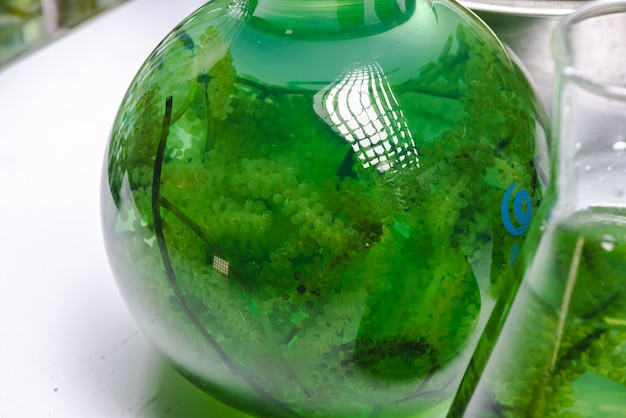The photograph appears to have been taken in a lab setting, featuring a variety of glassware on a white lab bench under reflective fluorescent lighting. Among the glassware, the main focus of the image is a large round-bottom flask, filled with water and containing a bright pea green aquatic plant. This plant has multiple spherical, grape-like protrusions along its stems, which are floating in the water. The flask, partially showcasing a blue manufacturer's logo, sits centered in the image. On the right edge of the photo, you can see part of a beaker, while additional glassware is visible in the background. The background consists of a white surface and a gray-green hue due to the reflection and lighting in the lab.